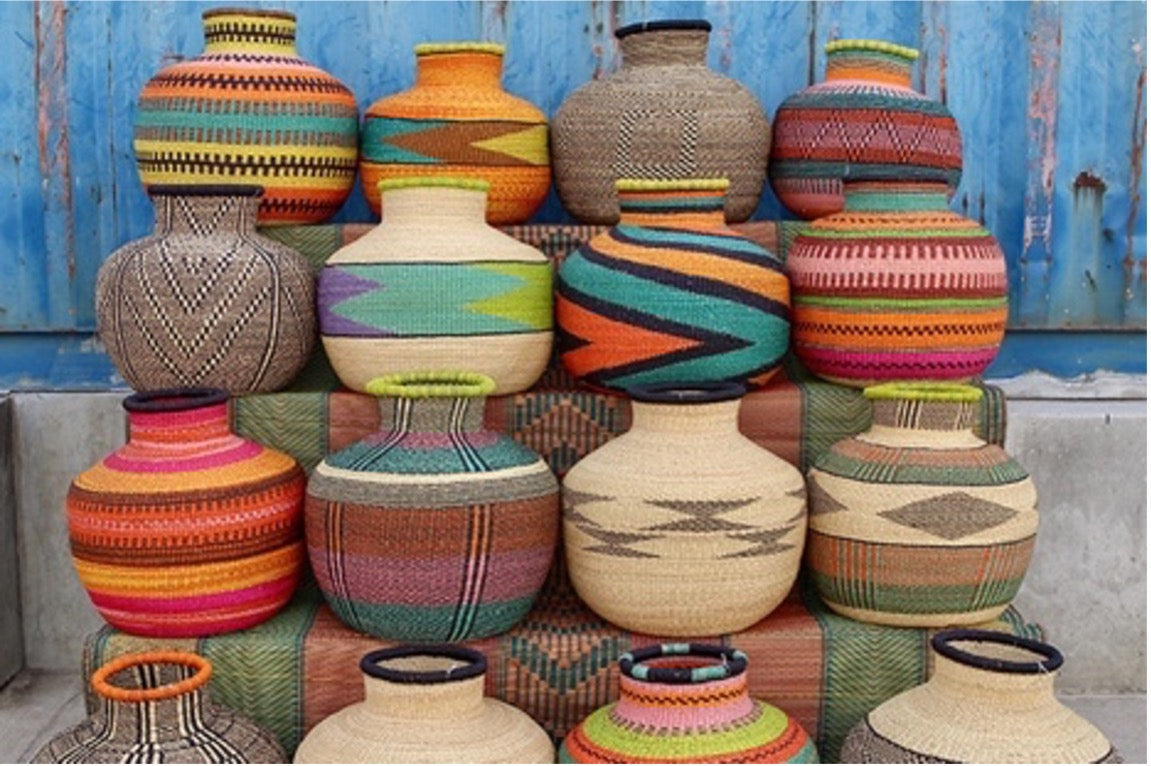This image captures a vivid display of 16 intricately crafted pots, skillfully arranged on outdoor stairs with four pots per step. The backdrop features weathered wood painted a rich blue, adding a rustic charm to the scene. These uniquely designed pots exhibit Native American or Aztec-inspired prints and boast a wide array of colors, including vibrant shades of orange, teal, pink, yellow, cream, blue, green, brown, and tan. The pots are made from a braided and knit fabric, giving them a textured appearance. Their shape is characterized by a wide base that tapers to a narrow top. While they appear robust and heavy, they are surprisingly lightweight due to their fabric construction. Whether meant for decorative purposes or as potential vessels for flowers, these eye-catching pots make a striking and colorful display with their diverse patterns and hues.